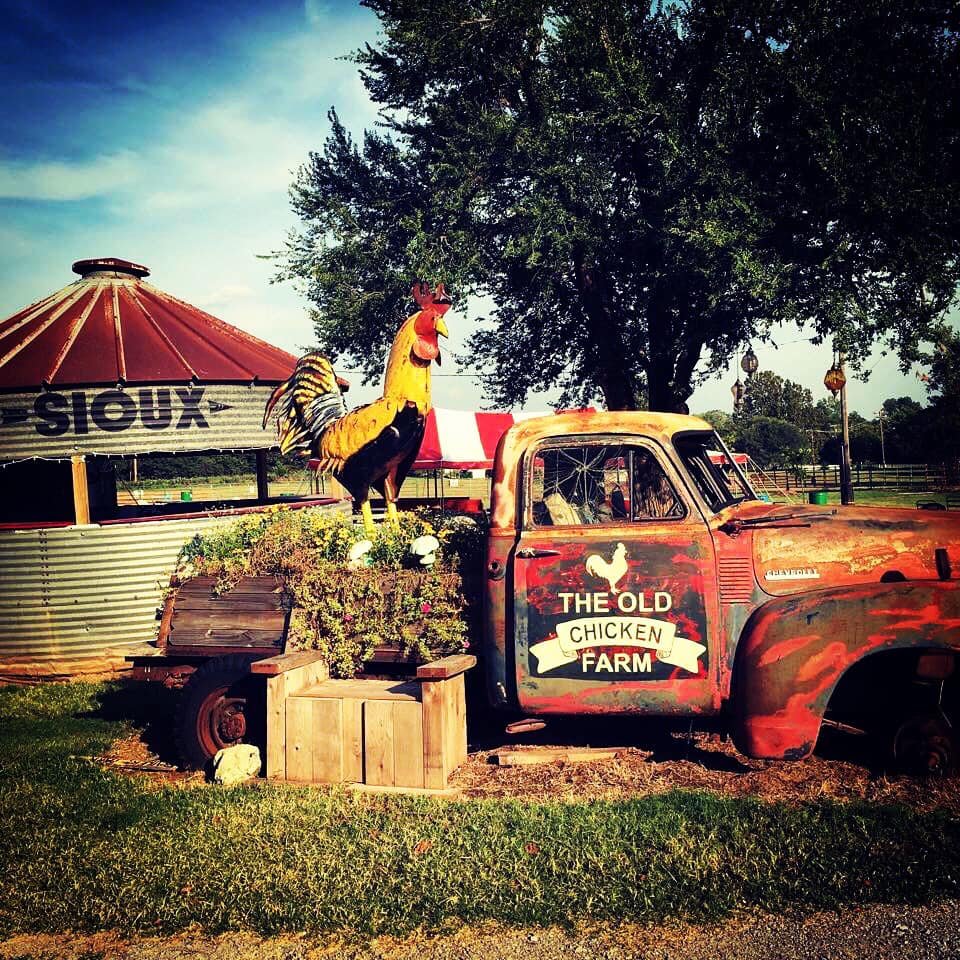In this scenic outdoor image, an old, colorful truck from the 1930s or 40s stands prominently in the foreground, repurposed as a garden bed filled with diverse foliage. The truck’s door bears the words "The Old Chicken Farm" along with a silhouette of a chicken against a red and black backdrop. A large yellow and black rooster figurine stands proudly among the plants in the truck's flatbed. Adjacent to the truck is a little wooden stand or bench adorned with vegetation. Behind the truck rises a short, metal structure with a red roof, labeled "Sioux." The lush surroundings feature green grass, a tall tree with full, green leaves on the right, and fences stretching into the background, hinting at a farm setting. Above, the sky transitions from a dark blue in the top left corner to lighter hues interspersed with white clouds, enriching the overall vibrant and bucolic scene.